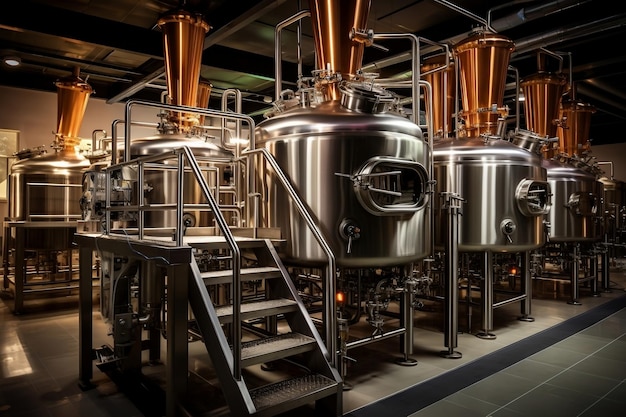The photograph captures a meticulously clean, indoor brewery or distillery, with a distinctly industrial aesthetic. The image showcases several large, cylindrical stainless steel vats, each topped with a copper-colored funnel or chimney attachment. These vats, raised off the concrete and tile floor on sturdy steel frames, are arranged in two visible rows. Steps and ramps provide access to oval glass doors on the vats, which offer a view inside. A walkway runs down the center for easy access to the tops of the vats. Various pipes and mechanisms are attached below each vat for drainage. The space is dimly lit by several industrial lights hanging from a dark-colored ceiling, highlighting the vats and casting a reflective sheen off of their polished surfaces. No personnel are visible in this highly organized production environment, which exudes a sense of precision and cleanliness, indicative of a facility dedicated to brewing or fermenting.